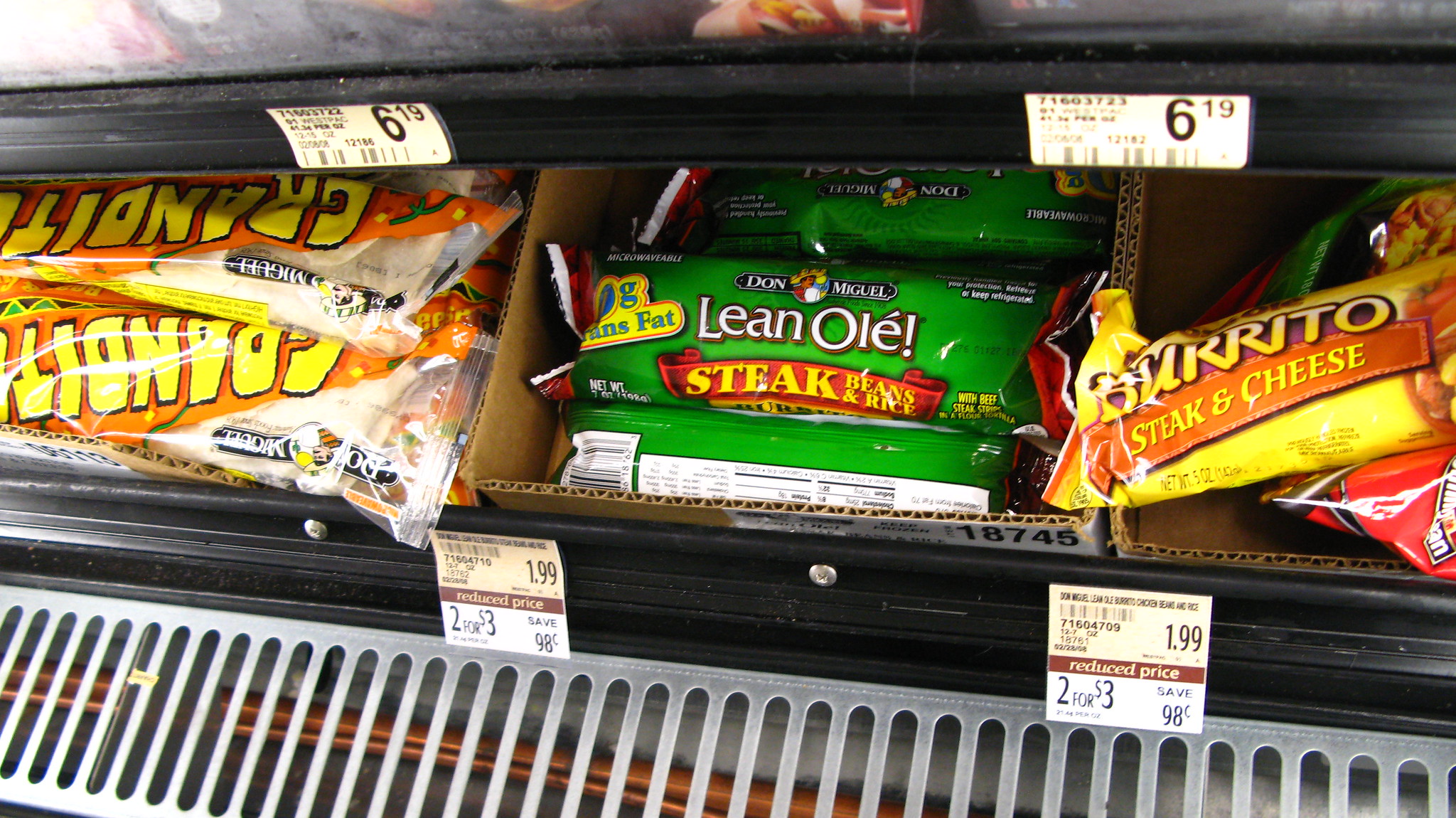The image depicts a refrigerated or frozen food section in a grocery store, primarily featuring a variety of packaged burritos. Each burrito is neatly arranged on black shelves and comes with clearly marked price tags. The burritos are packaged in different colors, with notable mentions of green, yellow, and red packaging. The green package, centrally located, shows Don Miguel burritos labeled "Steak, Beans, and Rice" with a price of $1.99 or two for $3.00, offering a saving of $0.98. burritos in yellow text are visible on another package, which advertises a burrito with steak and cheese. Additionally, there are identical price tags displaying $6.19, and another tag indicates a reduced price offer of $1.99 or two for $3.00. The burritos appear to be chilled, as evidenced by cold condensation on the packaging. The image also includes various price tags and product numbers such as 71653723. The overall scene showcases the organized display of burritos available for purchase in the frozen food aisle.